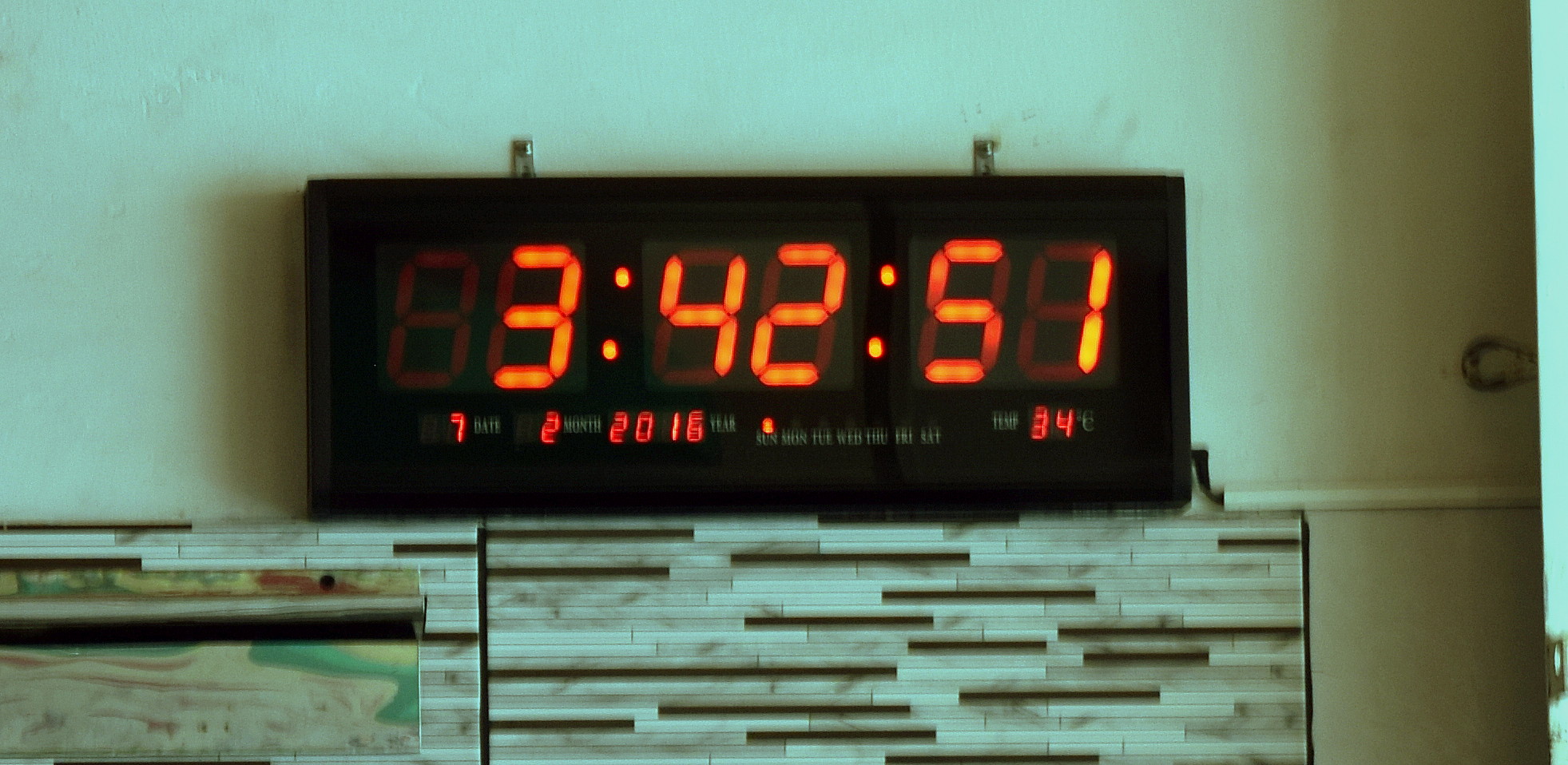The image depicts a large, black, rectangular digital clock, approximately five inches long, mounted on a wall with two visible tabs for support. The clock face displays the time in neon red numbers as "3:42:51." Below the time, additional smaller red numbers read "7 2 2016," indicating the date, along with the temperature "34°C" in the bottom right corner. The wall behind the clock features a backsplash composed of long, narrow tiles in a pattern of light brown, beige, and white horizontal rectangles. There's also a shadow cast on the right side of the clock. Additionally, in the lower left of the image, there appears to be a piece of artwork depicting abstract waves in beige, green, yellow, and red hues.